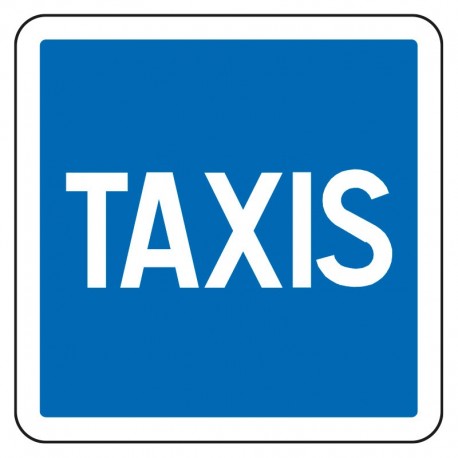The image depicts a square-shaped sign likely used for indicating taxi locations, such as near hotels or airports. The sign features a deep blue background framed by a white trim approximately an inch thick. Within this blue square, the word "TAXIS" is prominently displayed in tall, white, uppercase letters, possibly in a basic or Helvetica font. The sign's overall design is simple and straightforward, with clean, vertical lines in the lettering. While it appears visually as if it could be a digital creation or clip art rather than an actual photograph, it effectively communicates its purpose to direct both taxis and passengers efficiently.